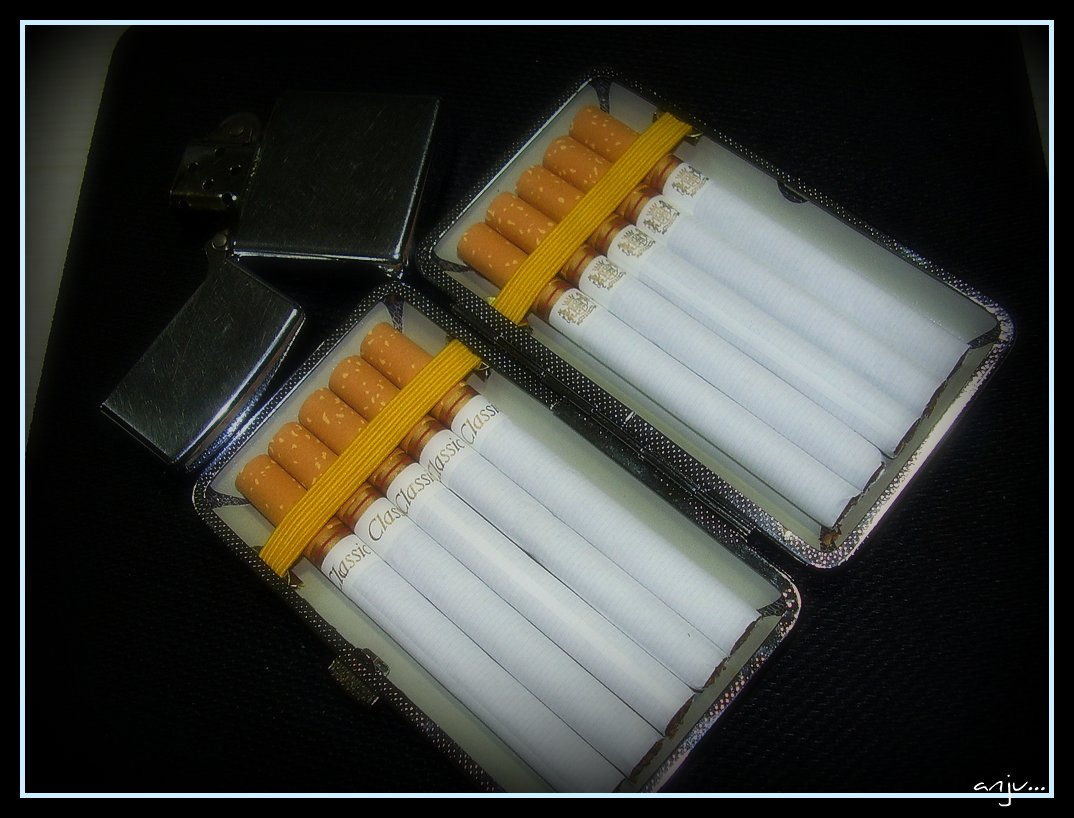This photograph captures a diagonally-oriented, silver cigarette carrying case opened up against a black fabric background. The case, resembling an open book, is positioned with its corners pointing from the bottom left to the upper right. It features a yellow band near the top securing 10 cigarettes in place, aligned five on each side. The cigarettes are white with brown filters and bear the label "classic" in gold lettering. Additionally, the left side of the case displays imaging on the cigarettes, though specific details are unclear. To the top left of the cigarette case sits an open Zippo lighter, with its cap fully hinged open. The image is set in a white inset frame and signed "ANJU..." at the bottom.